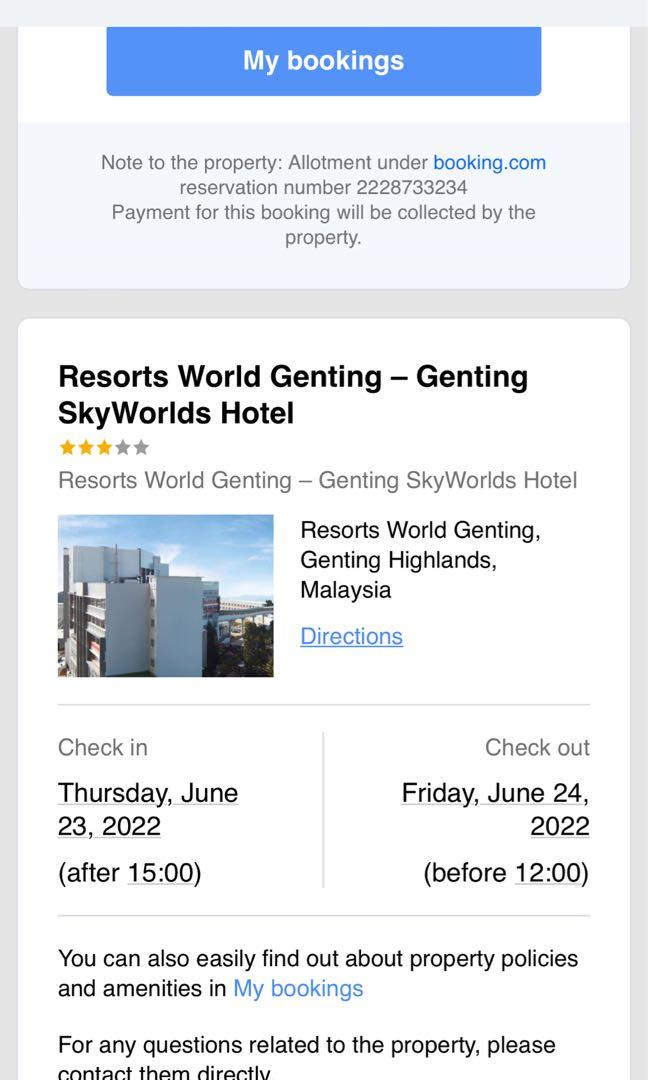This is a detailed screenshot depicting a hotel booking on a third-party website. The image is in portrait orientation, framed with a thin gray border along the top and sides. The top section features a white box with a long rectangular blue box inside, displaying the title "My Bookings" in white font. Below that, a grayish box contains information such as "Note to Property," "Employment under Booking.com," and "Reservation Number." It also mentions that the payment for this booking will be collected by the property.

Further down, a white rectangular box in portrait orientation displays the booking details in black font. The hotel name "Resorts World Genting, Genting Skyworks Hotel" is shown with a 3 out of 5 stars rating. Additional text repeats the hotel name and provides the location: "Resorts World Genting, Genting Highlands, Malaysia." To the left of this information is a small picture of the hotel and a blue link labeled "Directions."

A thin gray border separates this section from another box, which lists the check-in and check-out details. The check-in is scheduled for Thursday, June 23rd, 2022, after 15:00, and the check-out is on Friday, June 24th, 2002, before 12:00. Additional notes advise that property policies and amenities can be found in "My Bookings," and any property-related inquiries should be directed to the hotel.

This image clearly shows that the user is booking the hotel through a third-party website.